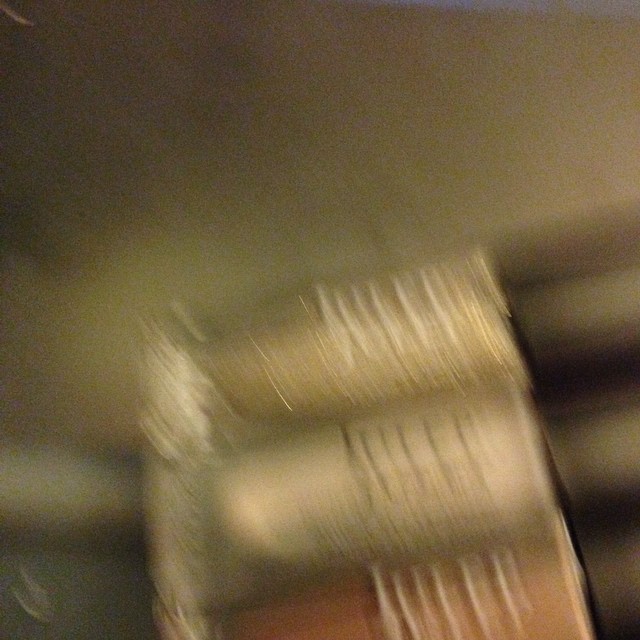In the image, a shadowed interior is portrayed, with the ceiling predominantly dark in the top left corner, transitioning into lighter brown and silver hues towards the side. On the left, several stark white rectangles catch the eye, contrasting sharply with a darker gray area at the bottom. The right side of the image is almost entirely white. 

Near the right, there appears to be a stack of items, somewhat blurry, with text on them. The first item has a yellowish tint and seems to spell "Juliet." The subsequent items are also labeled "Juliet," although the blur makes it difficult to decipher the words clearly. These items appear to be tubes or cylindrical objects, aligned vertically and seemingly attached to a wall on the left-hand side.